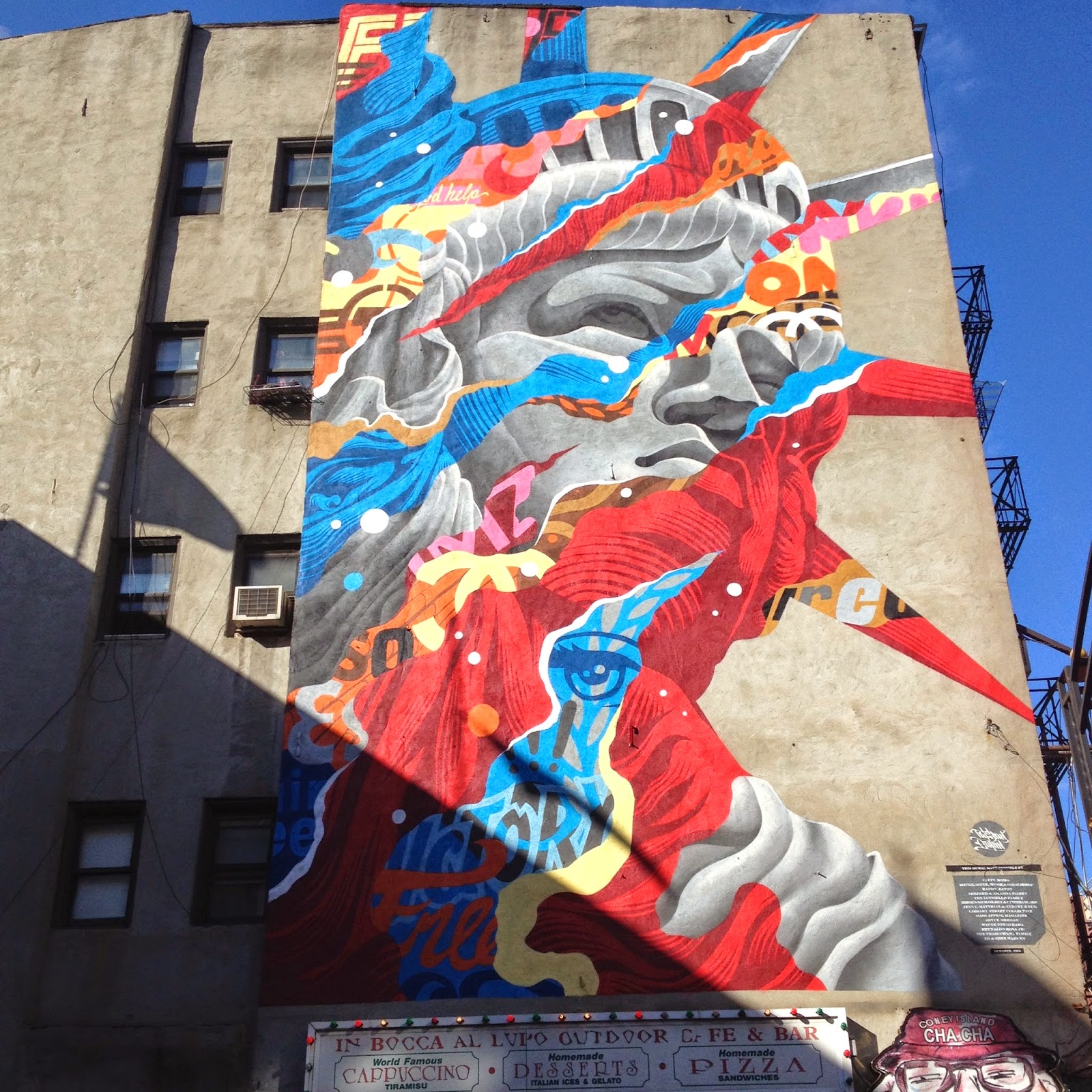This detailed photograph showcases an intricate mural painted on the side of a tall, old gray stone building, which appears to house apartments. The centerpiece of the mural is the Statue of Liberty, rendered in an alluring mix of blue, red, yellow, and other vivid colors, deviating from her traditional greenish hue. The mural employs a dynamic interplay of red, blue, and white lines flowing through Lady Liberty's face and crown, adding vibrancy and a modern twist to the classic icon. Notable details include a bird painted within the red section, featuring blue and yellow hues. The left side of the building features eight discernible windows, some with window air conditioning units, while the right side reveals balconies or fire escapes against a backdrop of blue sky. A triangular shadow is cast upon the left corner of the mural, adding depth to the visual. Below the Statue of Liberty, an advertisement reads "In Boca El Outdoor Cafe and Bar Cappuccino Pizza," indicating the presence of a cafe or pizzeria at street level.